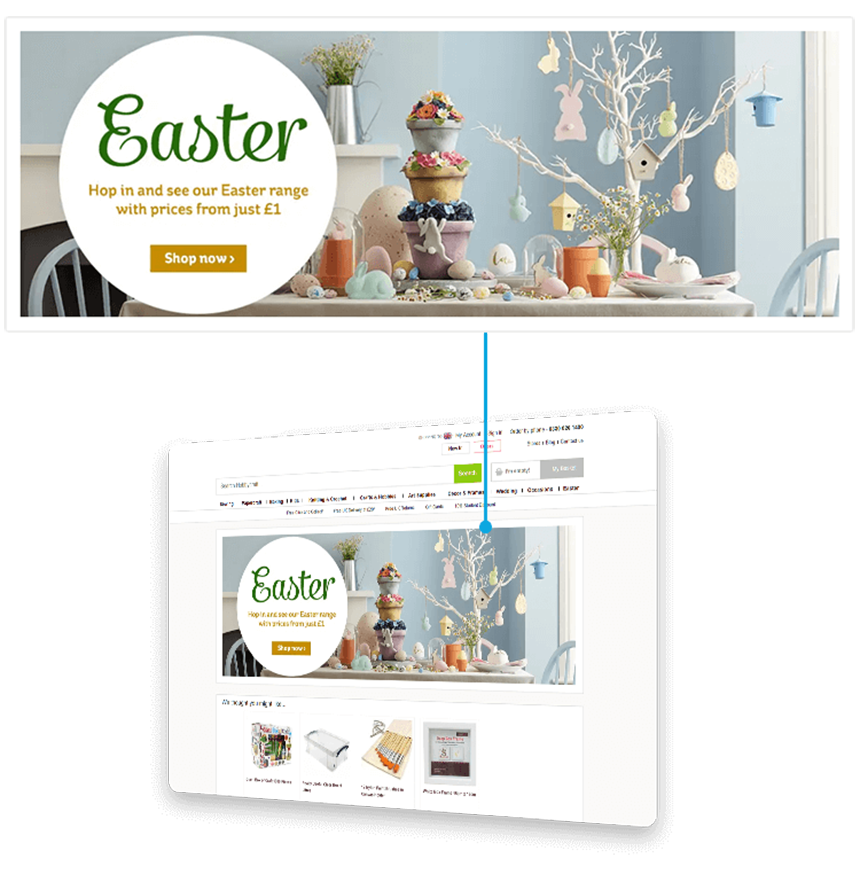The image is a promotional advertisement divided into two distinct parts. The focal point of the bottom section is a computer screen, depicted in a three-dimensional rotation, making the right side appear closer to the viewer than the left. The screen itself is white and prominently features a circular banner with the word "Easter" and an accompanying advertisement. This detailed screen shot includes various elements like multiple tabs, and a rectangular segment at the bottom highlighting four items available in a store.

Connecting the screen to the top part of the image is a blue line ending in a small circle. This links to a magnified version of the Easter banner in a two-dimensional format. The banner's text is shown in green and gold, reading, "Easter" in green, followed by "hop in and see our Easter range with prices from just £1. Shop now" in gold.

In the background of the scene is a table with two chairs set against a robin’s egg blue wall, creating a cozy atmosphere. The setting is adorned with Easter-themed decorations, including a white sculpture of a small tree festooned with various hanging ornaments such as bunnies, houses, and eggs. Additionally, a charming sculpted bunny is pictured climbing a series of flower pots, each stacked within the other. The overall scene effectively highlights and promotes the Easter-themed advertisement.